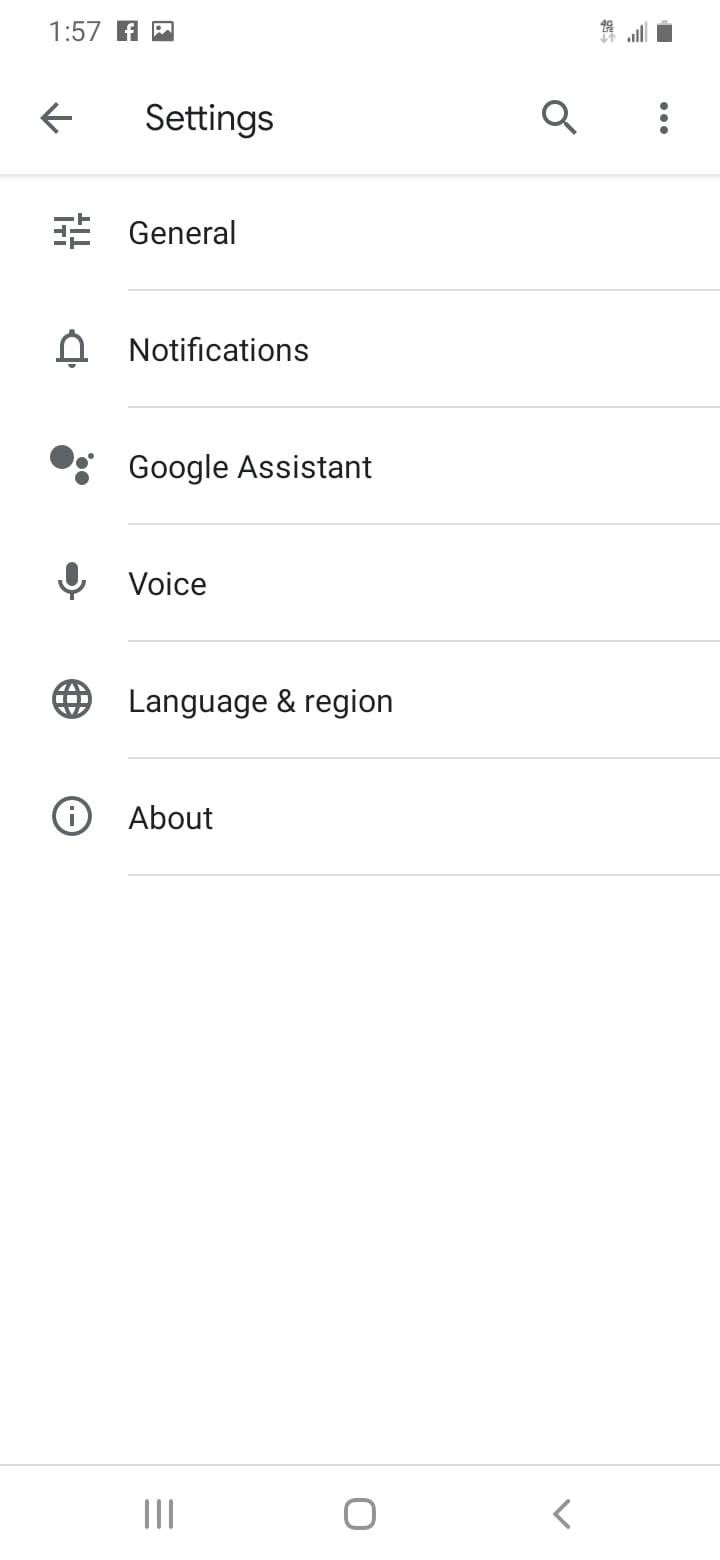Screenshot of a phone with a white background displaying a timestamp of 1:57. The upper section shows various status icons, including a Facebook icon and signal strength indicating 4 out of 5 bars, among other unclear icons. Below this, there's an arrow pointing left, next to the word "Settings," followed by a magnifying glass icon and a vertical ellipsis. 

Beneath a gray horizontal line, the "General" option is listed with an indiscernible icon to its left. Following that, another horizontal line appears. Next, a bell icon denotes the "Notifications" setting. Further down, an icon resembling a cluster of circles represents the "Google Assistant" option, followed by another dividing line. Below this, a microphone icon signifies the "Voice" setting, separated by yet another line. Subsequently comes a globe icon labeled "Language and Region," with another dividing line after it.

Near the bottom, there's a white oval containing a lowercase "i," situated to the left of the "About" section text.